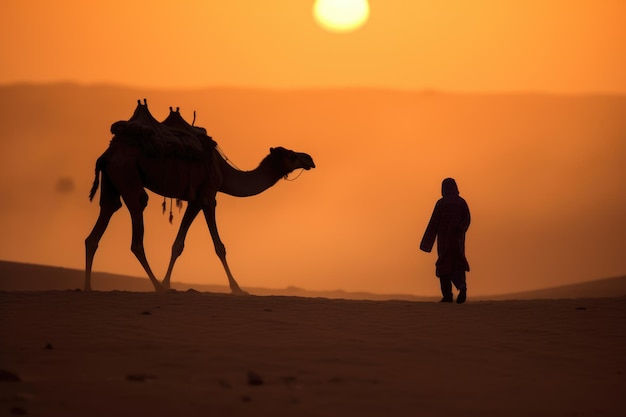The image depicts a stylized and dramatized outdoor desert scene at sunset. The landscape foreground is characterized by a sandy or dusty floor in dark brown hues, smoothly transitioning to a bright orange midsection and topped off by a yellow gradient that fades into the sky. A small, bright yellow sun is visible, low on the horizon, suggesting a setting sun. The scene features two shadowy figures rendered in black silhouette: on the right-hand side stands a person, and on the left-hand side, a camel adorned with two saddles, one over each hump. The figures are in stark contrast to the colorful, muted background, contributing to the hazy and atmospheric quality of the twilight desert setting.